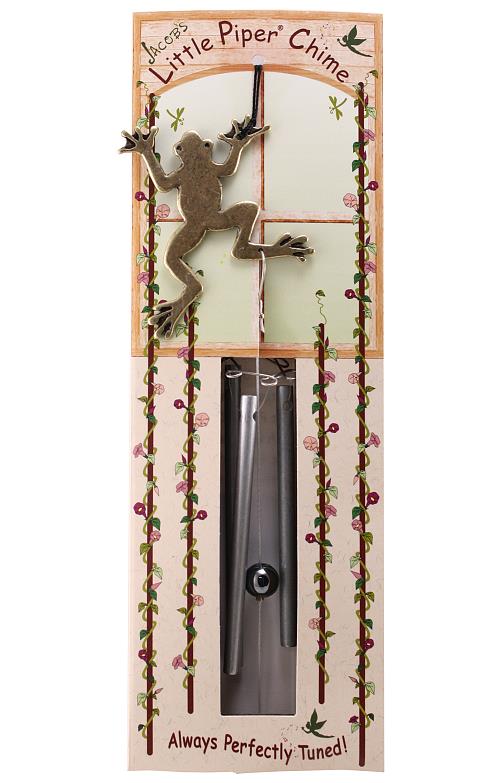The image showcases a pink rectangular cardboard package for a wind chime, prominently labeled at the top with "Jacob's Little Piper Chime" in red and brown text. The packaging features detailed illustrations, including a brown frog with large webbed feet appearing to climb down the chimes, and four long brown sticks adorned with vines and pink and purple flowers. A cut-out window reveals the actual silver, hollow wind chimes, with a central silver ball hanging from a string. At the bottom of the package, the text "Always Perfectly Tuned" is prominently displayed in red, emphasizing the quality of the product. Overall, the decorative design and the peek into the product inside give a charming and whimsical preview of the wind chime.